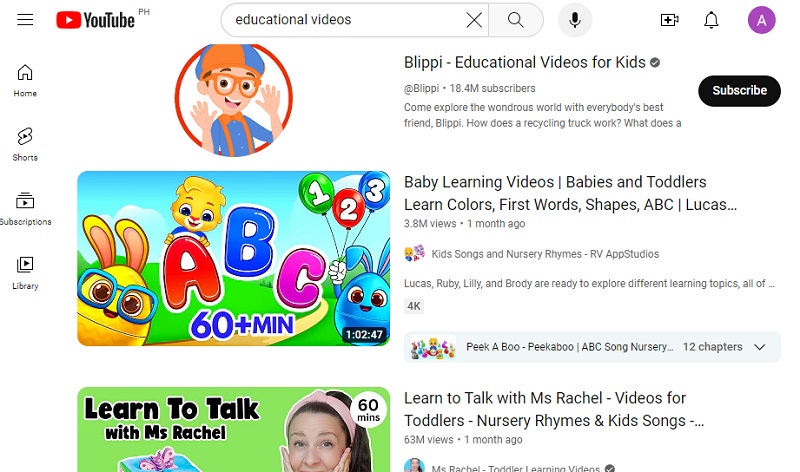This is a detailed screenshot of the YouTube interface. At the top left, there are three horizontal bars representing the menu. Moving to the right, the iconic YouTube logo with its red play button is prominently featured. The central area of the interface has a search bar where the term "educational videos" is typed, accompanied by a circular 'X' button for clearing the search. A magnifying glass icon for initiating a search is positioned next to the search bar. Adjacent to these elements is a circle embedding a microphone symbol, allowing for voice search functionality. Following this, there are icons for the camera, notifications, and a profile picture placeholder on the top right, which notably includes a purple button with the user's first initial.

Scrolling down to the search results, the first entry features Blippi, a vibrant cartoon character known for educational content. Blippi is depicted as a young boy wearing orange glasses, an orange and blue outfit, with his hands raised joyfully and a big smile aimed at the viewer. Below Blippi, there are several thumbnails showcasing other educational content for children. These include types of learning videos for babies and toddlers, covering topics such as learning colors, first words, shapes, the alphabet, and featuring characters like Lucas and various animated animals. The titles continue with options such as "Learn to Talk with Ms. Rachel," "Videos for Toddlers," and collections of nursery rhymes and kids songs—all listed vertically.

In one specific thumbnail below Blippi, there is an array of cartoon characters including a yellow rabbit, a blue rabbit, and another yellow character standing near an 'ABC' sign, contributing to the motif of colorful, educational themes aimed at young learners.